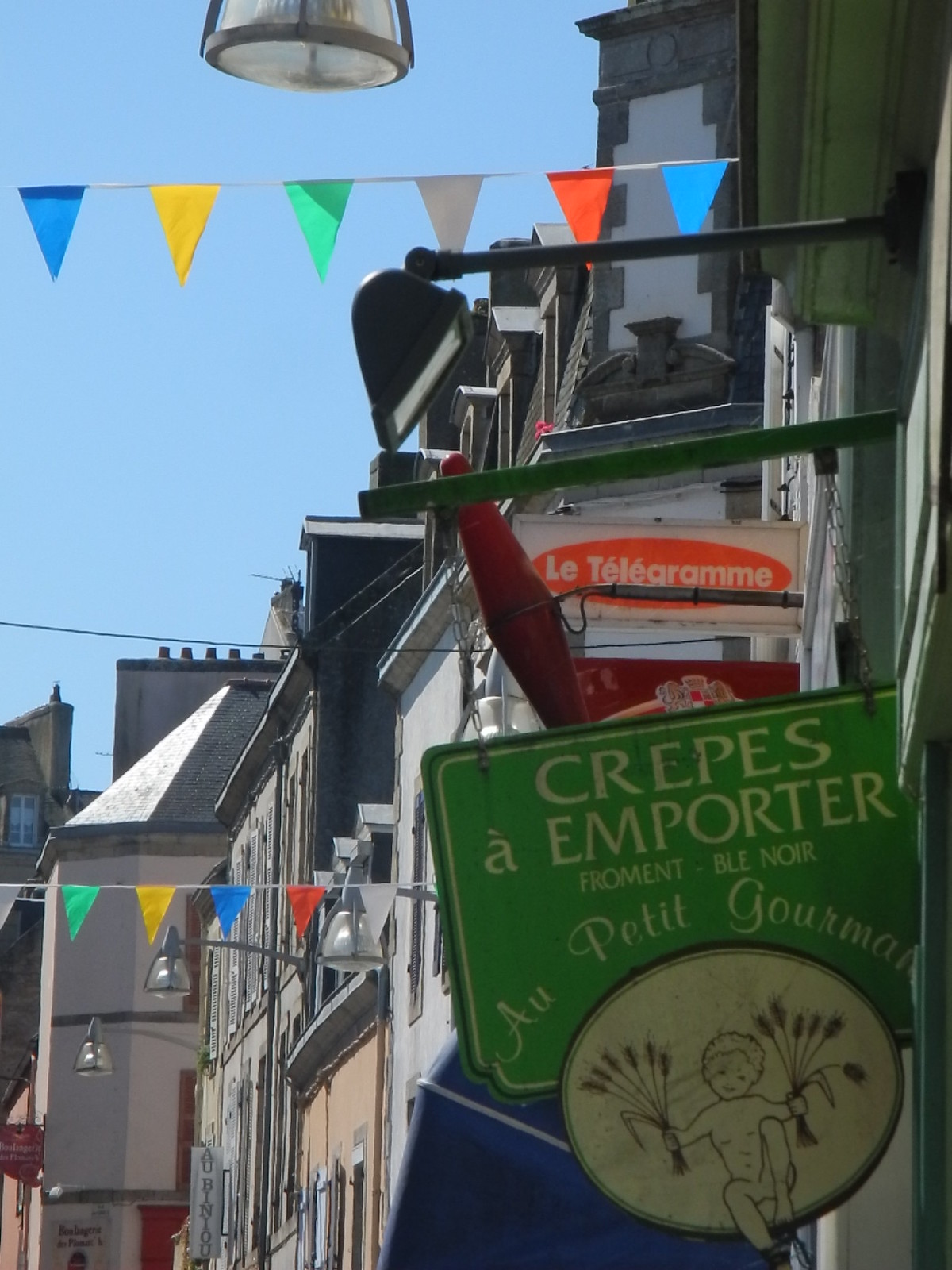In this vibrant street scene, a plethora of signs and banners adorn the facades of gray buildings. Positioned in the lower right half of the image is a somewhat weathered green sign with white lettering, proclaiming "Crepes Importer." Below this, the text reads "Au Petit Gourmand." The sign also features a circular emblem extending below its bottom edge, depicting a white silhouette of a boy holding strands of flowers in both hands. Directly beneath this sign is a blue awning projecting outward. Above the bustling street, an array of colorful pennants—blue, yellow, green, gray, red, and blue again—sway gently, strung across the road, adding to the festive atmosphere. More buildings further down the street are similarly adorned with these spirited pennants, contributing to the lively, celebratory vibe. A light fixture hangs down from the top of the frame, casting a warm glow on the scene below. The blue sky serves as a perfect backdrop, enhancing the lively, market-like setting where stores exhibit their offerings, suggesting a local festival or cultural event.